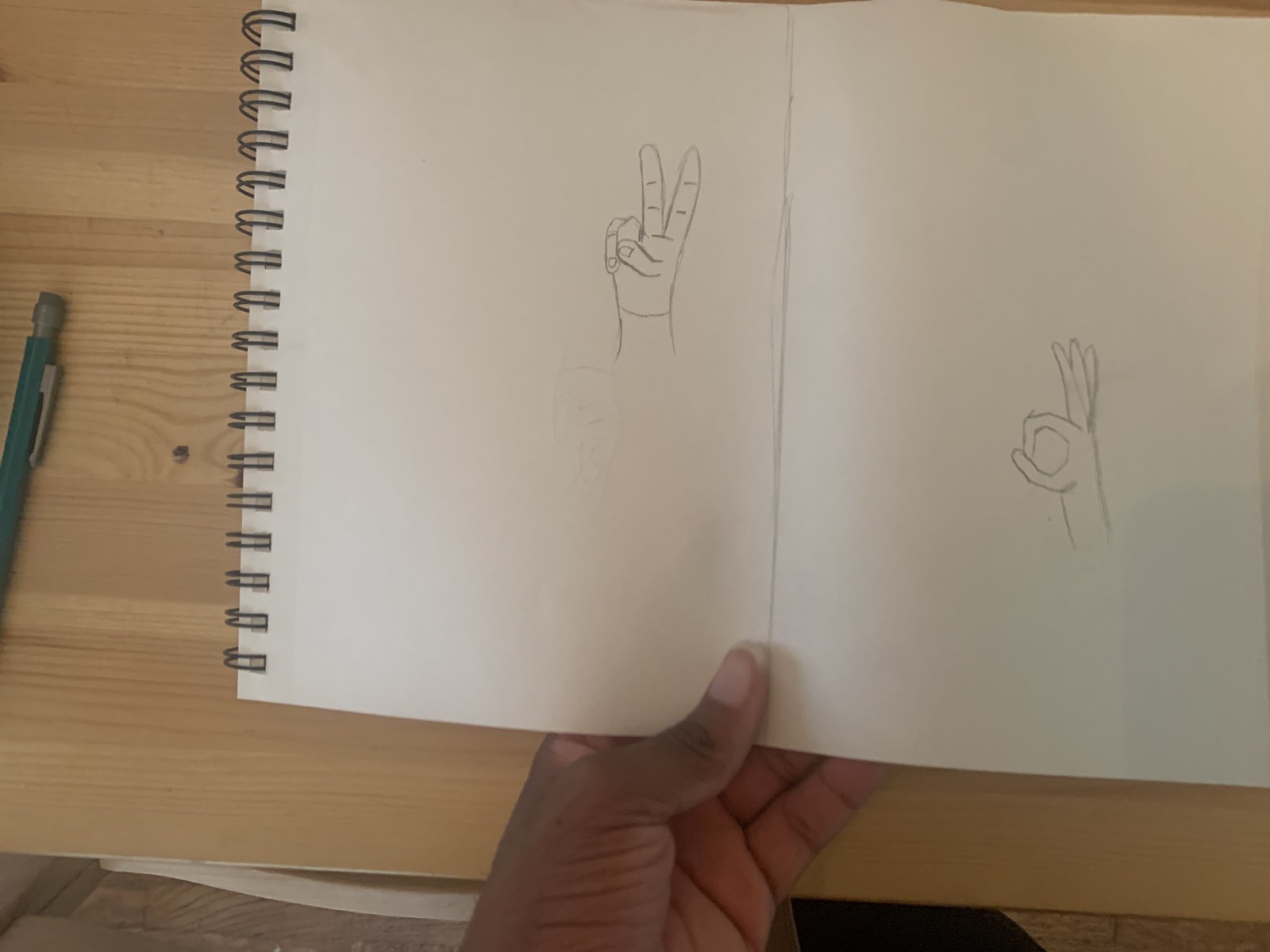The image showcases a long, white notepad bound with black rings, lying open on a light brown wooden tabletop. In the center of the notepad, a detailed pencil drawing depicts two hand gestures. On the left side of the page, a hand is making a peace sign, with the index and middle fingers raised and the remaining fingers folded down. To the right of this, another hand is forming an "okay" gesture, with the thumb and index finger touching to create a circle, while the other three fingers are pointed upwards. A green mechanical pencil with a brown cap rests on the table to the left of the notepad. A dark brown-skinned hand holds the notepad open, its palm and thumb partially visible under the paper. The setting appears to be a casual environment, potentially a classroom or home desk, with a glimpse of brown flooring visible at the bottom of the image.